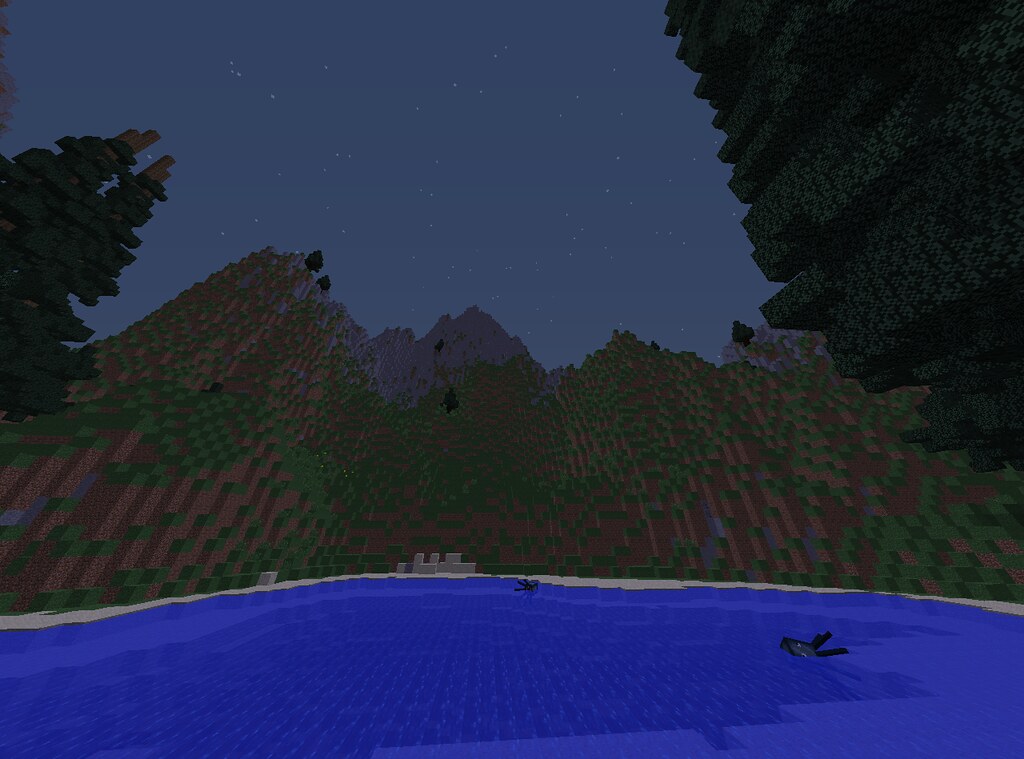The image appears to be a screenshot from the pixelated video game Minecraft. At the top of the image, the sky transitions into a very dark gray, suggesting it is nighttime. Twinkling stars are visible against the computerized sky. In the background, there are silhouetted mountains, partially framed by the edges of trees. Moving into the midground, a blue lake stretches across the scene, creating a serene contrast to the dark sky. In the lake, there are two individuals who look like they might be swimming. These figures are not detailed but appear blocky, characteristic of the game's style. At the base of the mountains, just behind the lake, a few small, blocky, gray buildings are nestled, adding a sense of civilization to the otherwise natural landscape.